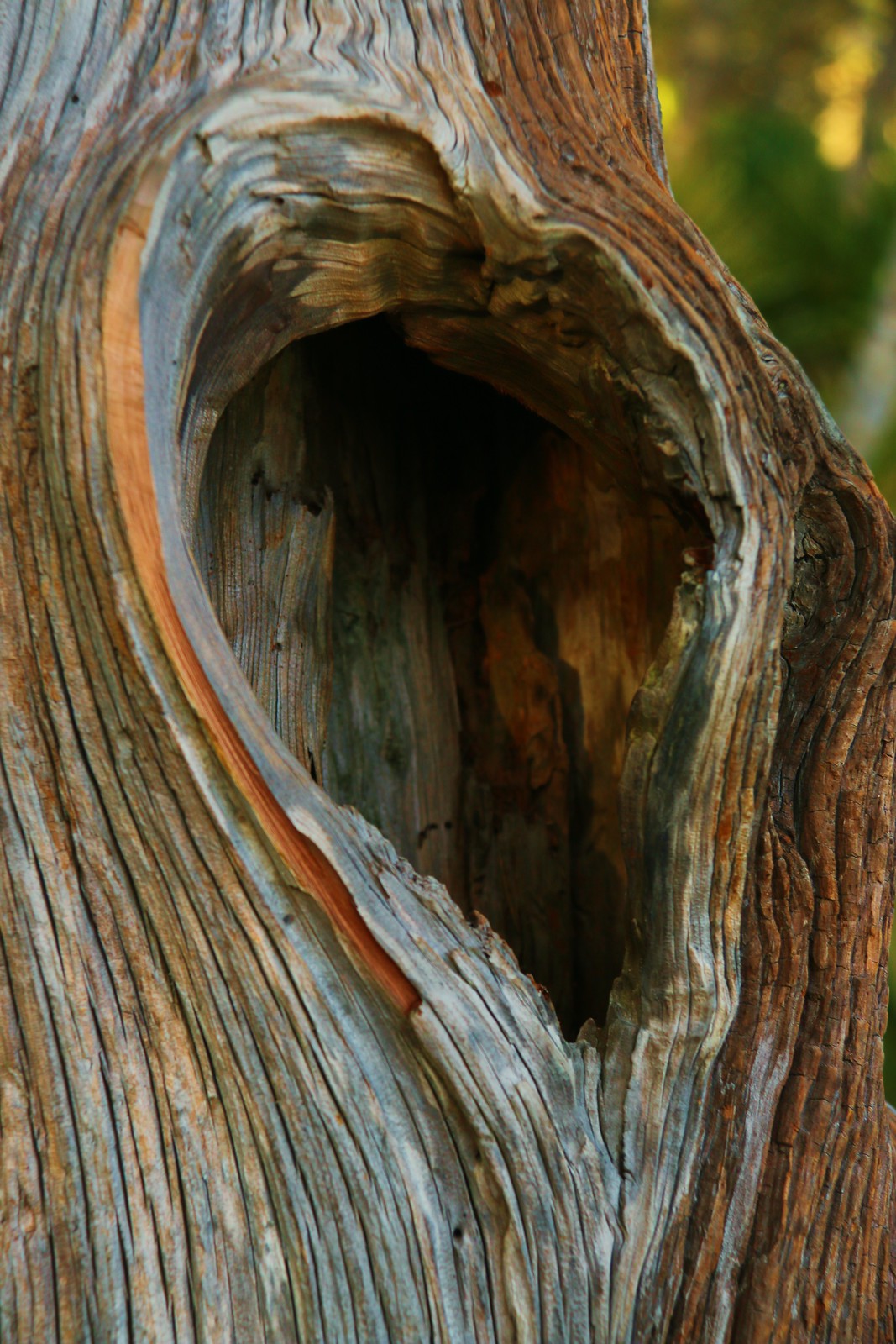This detailed close-up photograph captures a tree stump featuring a sizable hole, shaped like an upside-down heart or pear. The surrounding bark appears faded and aged, with a texture that includes vertical striations and cracks, suggestive of rot. The tree itself is a light grayish-tan color and looks like an old, possibly dead, specimen situated in well-watered ground. The hole, approximately 6 to 12 inches in size, extends deeply into the tree, offering a glimpse into a darker interior. Nothing currently occupies the cavity. In the blurred background to the upper right, some greenery can be seen, illuminated by fading evening light, adding a subtle touch of late-day ambiance to the scene.